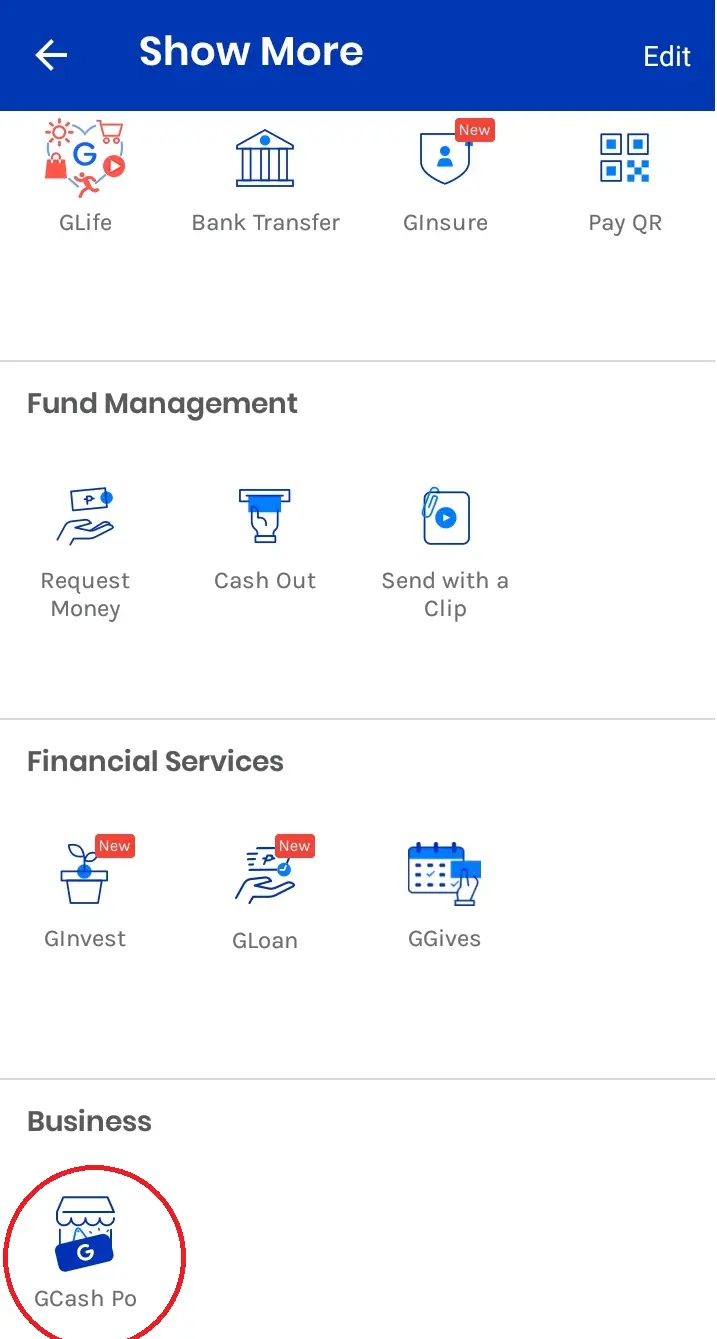Here is a detailed and clean caption for the screenshot of the financial app:

---

Screenshot of a financial app interface, likely a banking application. At the top, there is a blue navigation bar featuring a white back arrow on the left, a "Show More" label, and an "Edit" option on the right. Below the navigation bar, there are four main icons with accompanying labels:
- A heart icon labeled "GLifeUnder."
- A building with columns labeled "Bank Transfer."
- A shield icon labeled "GInsure."
- A QR code labeled "PayQR."

A horizontal line separates this section from the next. The subsequent segment is titled "Fund Management" and includes three options: "Request Money," "Cash Out," and "Send with a Clip."

Another dividing line follows, leading to the "Financial Services" section, containing "GInvest," "GLoan," and "GGives."

The final section, labeled "Business," features "GCashPO," which is highlighted with a red circle.

---